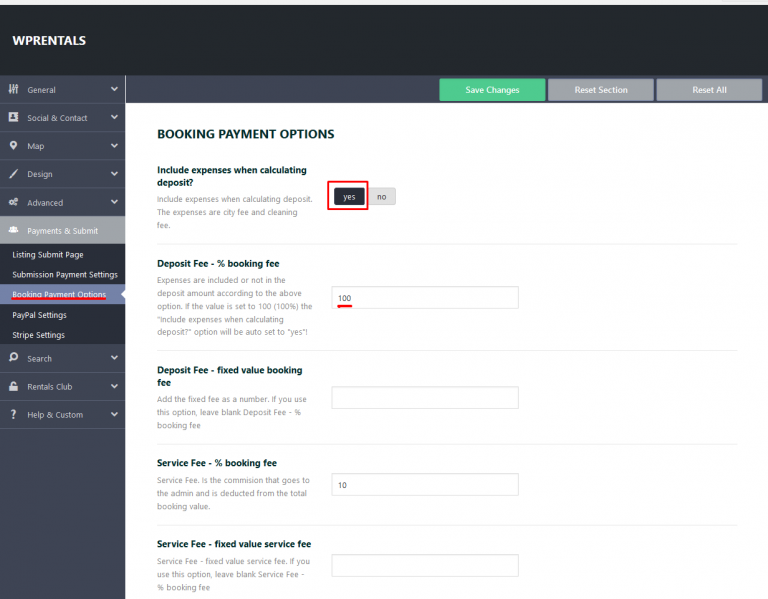The image depicts a screenshot of a computer screen displaying the "WP Rentals" interface. At the top, "WP Rentals" is prominently written in white text against a dark gray background. The left sidebar features several navigational options on a gray background: General, Social, and Contact, which are all drop-down menus. Additional options include Map, Design, Advanced, Payment, and Submit, with the latter being grayed out, indicating the current page is selected.

From the "Submit" drop-down are several sub-options listed: Listing, Submit Page, Submissions, Payment Setting, and Booking Payment Options. "Booking Payment Options" is highlighted and underlined in red, denoting the active selection. Below, there are further options such as PayPal Settings, Stripe Settings, Search, Rentals Club, Help, and Custom.

Within the "Booking Payment Options" section, the image features specific settings:
- "Include expenses when calculating deposit" with a choice between "Yes" or "No," highlighted with "Yes" encased in a red box.
- "Deposit fee percent booking" set at 100%, again underlined in red.
- "Deposit fee fixed value booking" is left blank.
- "Service fee percentage booking" is set at 10%.
- "Service fee fixed value service" remains unentered.

At the top of the screen, several action options are visible: "Save Changes," "Reset Selection," and "Reset All."